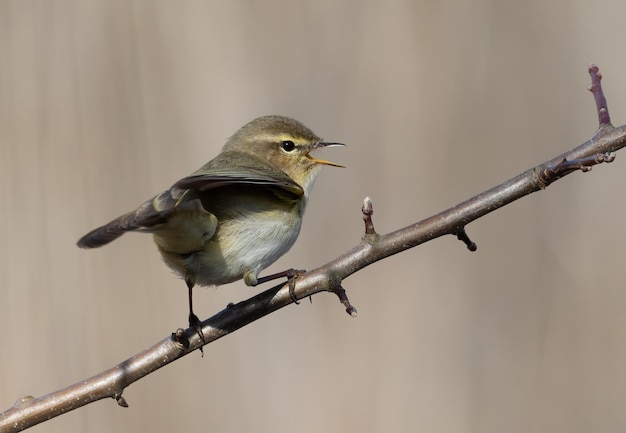This detailed image showcases a small bird, possibly a finch, perched on a budding branch, suggesting late winter or early spring. The branch, brown in color, extends diagonally from the lower left corner of the photograph towards the upper right, with several shorter offshoots. The bird, poised with its beak open as if chirping and eyes looking to the right, appears ready to take flight. It features a distinct coloration with shades of brown: lighter beige-white underbelly, darker brown feathers, a medium brown fuzz on its head, and yellow highlights around its eyes and beak. The background is a completely washed-out blend of tans, beiges, and grays, making the bird and the branch the clear focal points of the image.